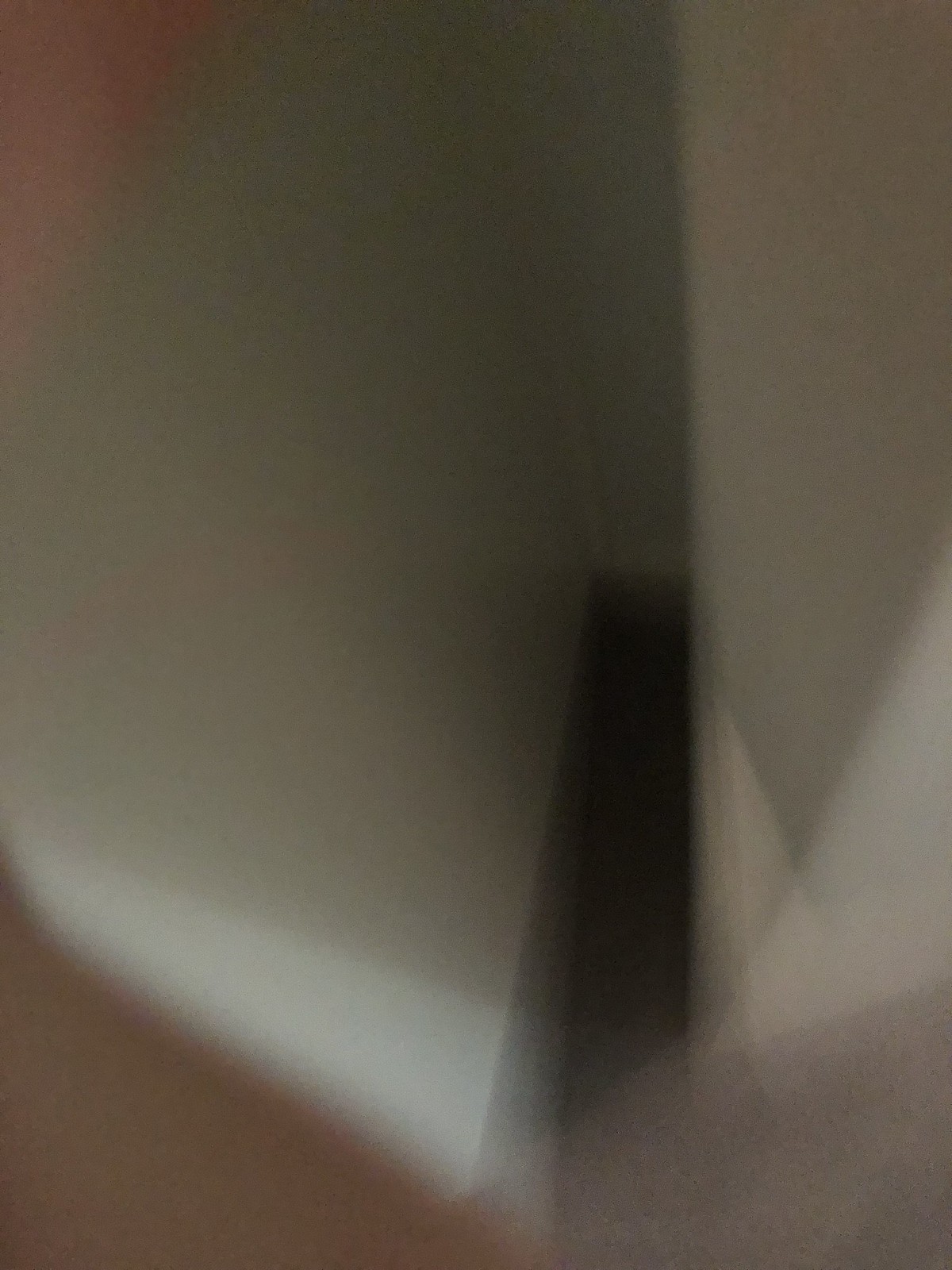The image depicts a highly blurry and abstract scene dominated by a central black rectangular shape that extends toward the bottom, creating a sense of depth. Surrounding this dark rectangle are varying shades of white and gray shapes, which become darker near the back and lighter towards the front, adding to the perception of depth. The bottom left corner features a slight yellow or reddish blur, transitioning to a larger diagonal brownish blur, which is adjacent to a lighter gray or triangular white shape above it. The right side of the image is predominantly beige with subtle shadows. Despite its abstract nature, the image evokes a feeling of looking down into a narrowing, shadowy space, possibly resembling a stairwell or a digital abstract art piece.